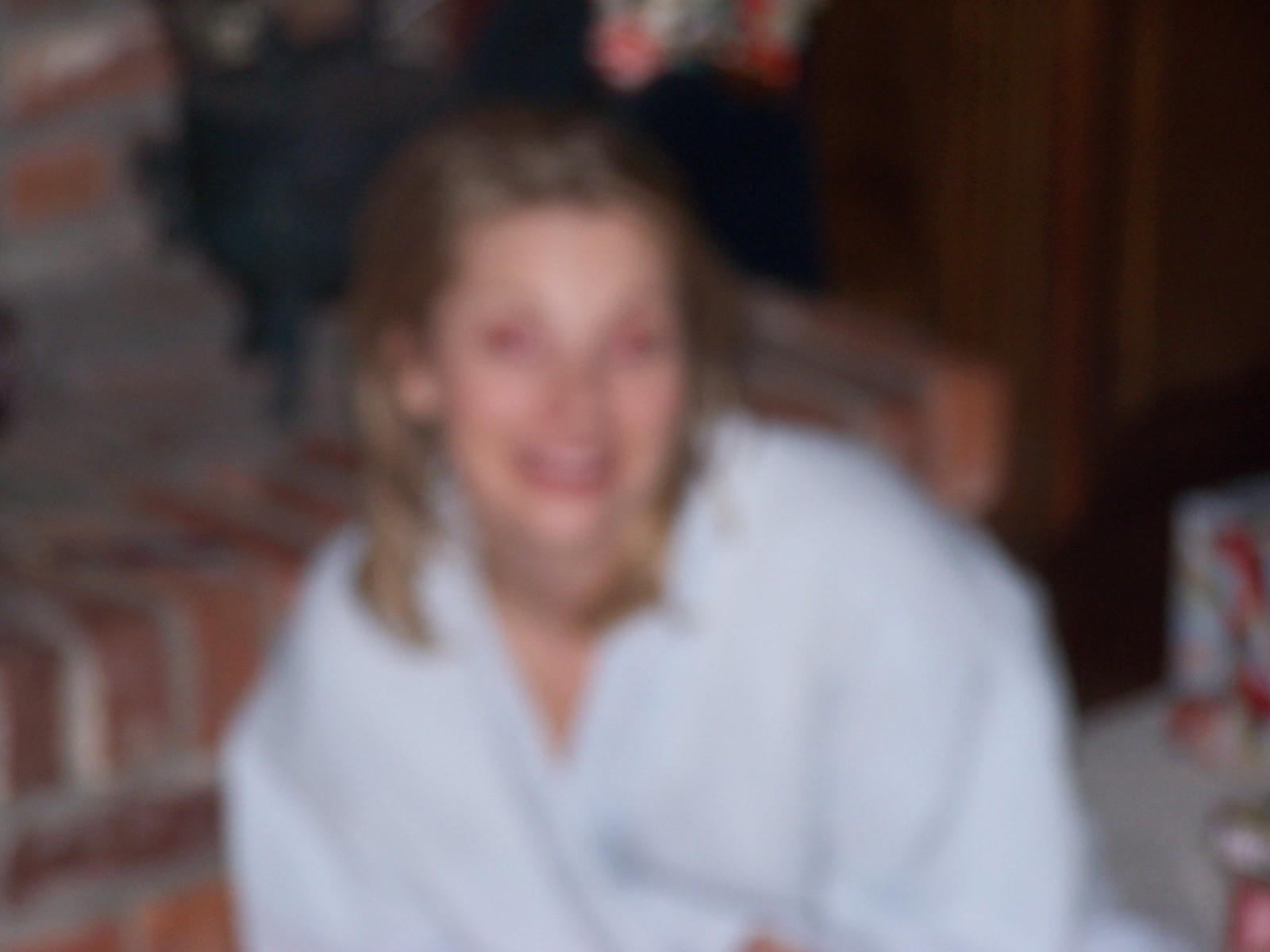In this very blurry image, a young woman with shoulder-length blonde hair is smiling directly at the camera. She appears to be wearing a white garment, possibly a sweatshirt, coat, or shirt. The setting seems to be indoors, as she is seated in front of a brick fireplace with white grout. The details inside the fireplace are not visible. The right side and the top area surrounding the woman are enveloped in a dark grayish-green color, with some indistinguishable white elements scattered throughout. There also seems to be tan carpet beneath her. The background might contain a Christmas tree, but it is too unclear to confirm. Overall, despite the image's blurriness, the cozy, indoor setting is discernible.